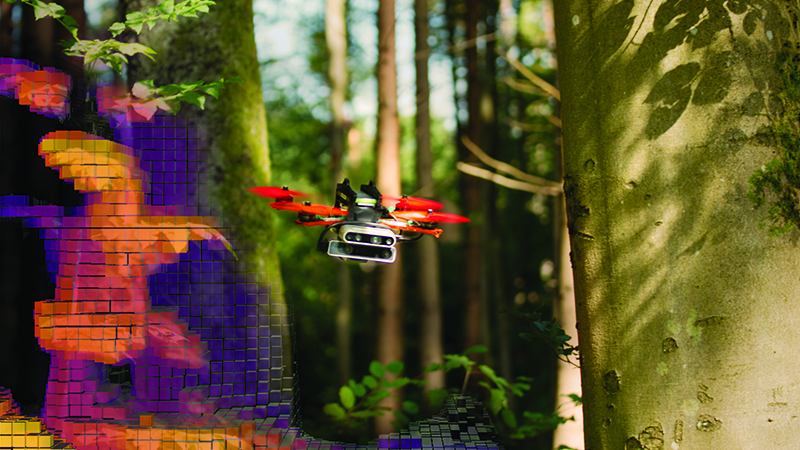In this surreal, outdoor image captured in a forest setting, a sleek black-framed drone with four whirring red propellers and a tri-lens camera hovers prominently in the air. The scene around the drone presents a juxtaposition of reality and digital artistry. On the right, natural elements dominate with several tree trunks in green and brown hues, branches, and leaves creating a typical woodland backdrop. However, the left side of the image deviates into an otherworldly vision where a tree seems to morph into a pixelated, multicolored mosaic of small, square blocks in shades of purple, orange, yellow, red, and blue, giving the impression of a 3D-generated, augmented reality effect. The blending of the natural and the artificial elements enhances the image's overall unreal and intricate quality.